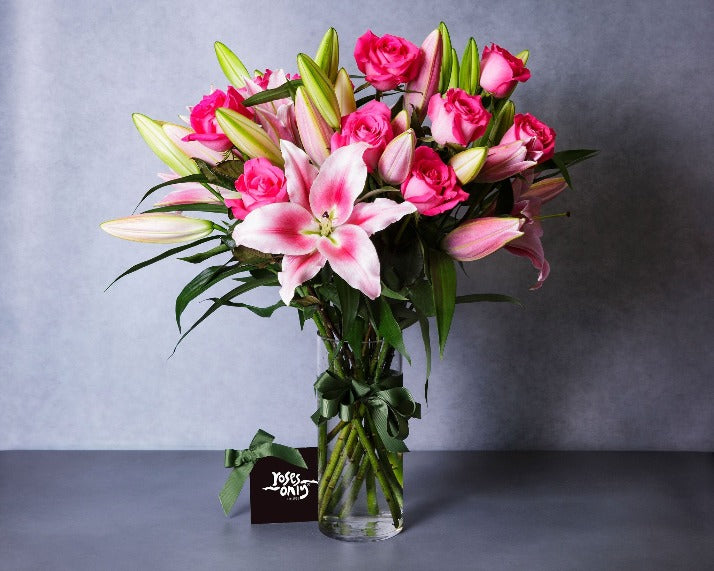The close-up image depicts a vibrant bouquet of flowers arranged in a clear glass vase, which is adorned with a picturesque green bow. The vase rests on a dark gray tabletop set against a muted grayish-blue background. The floral arrangement features a mix of pink roses and lilies, accompanied by lush green leaves. The flowers have thick green stalks that crisscross within the water-filled vase. While many of the roses are fully bloomed, the lilies are primarily closed, with a notable exception of a fully open pink and white lily at the front center of the bouquet. Accents of light green interior and smaller purple flowers add depth to the composition. 

To the left of the vase, there is a distinctive black tag that bears the white text "Roses Only," flanked by a white line extending horizontally on each side. The tag itself features a green ribbon tied to it. The arrangement includes both dark and light green leaves interspersed among the flowers, adding to the overall lush and vibrant appearance of the bouquet.